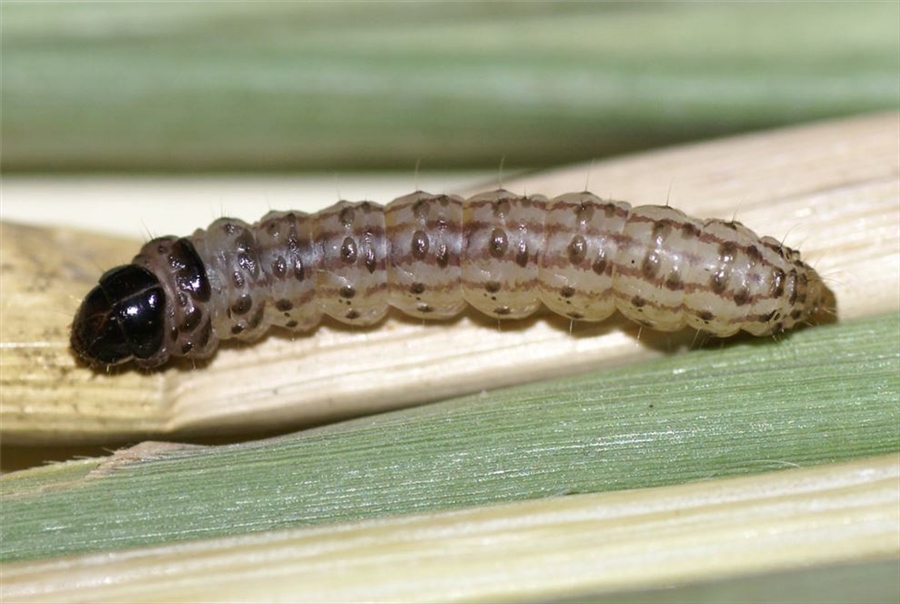In this highly detailed close-up photograph, the focus is on a caterpillar with a distinctly black head. The caterpillar's body is a light grayish-brown, somewhat reminiscent of a gummy bear texture, adorned with darker brown horizontal stripes and dots running down its back. Tiny, scarcely visible white hairs protrude from each body segment. The creature is lying horizontally on what appears to be a broad and flat pale brown leaf or branch, stretching almost entirely from the left to the right edge of the frame. The surroundings are well-lit, suggesting it's outdoors in natural light, though an external light source is also a possibility. Green leaves are present both in the foreground and background, with the backdrop being slightly out of focus, creating a soft blur that accentuates the caterpillar's intricate details. The caterpillar appears to be simply resting on the plant structure, offering a vivid and close examination of its unique physical characteristics.